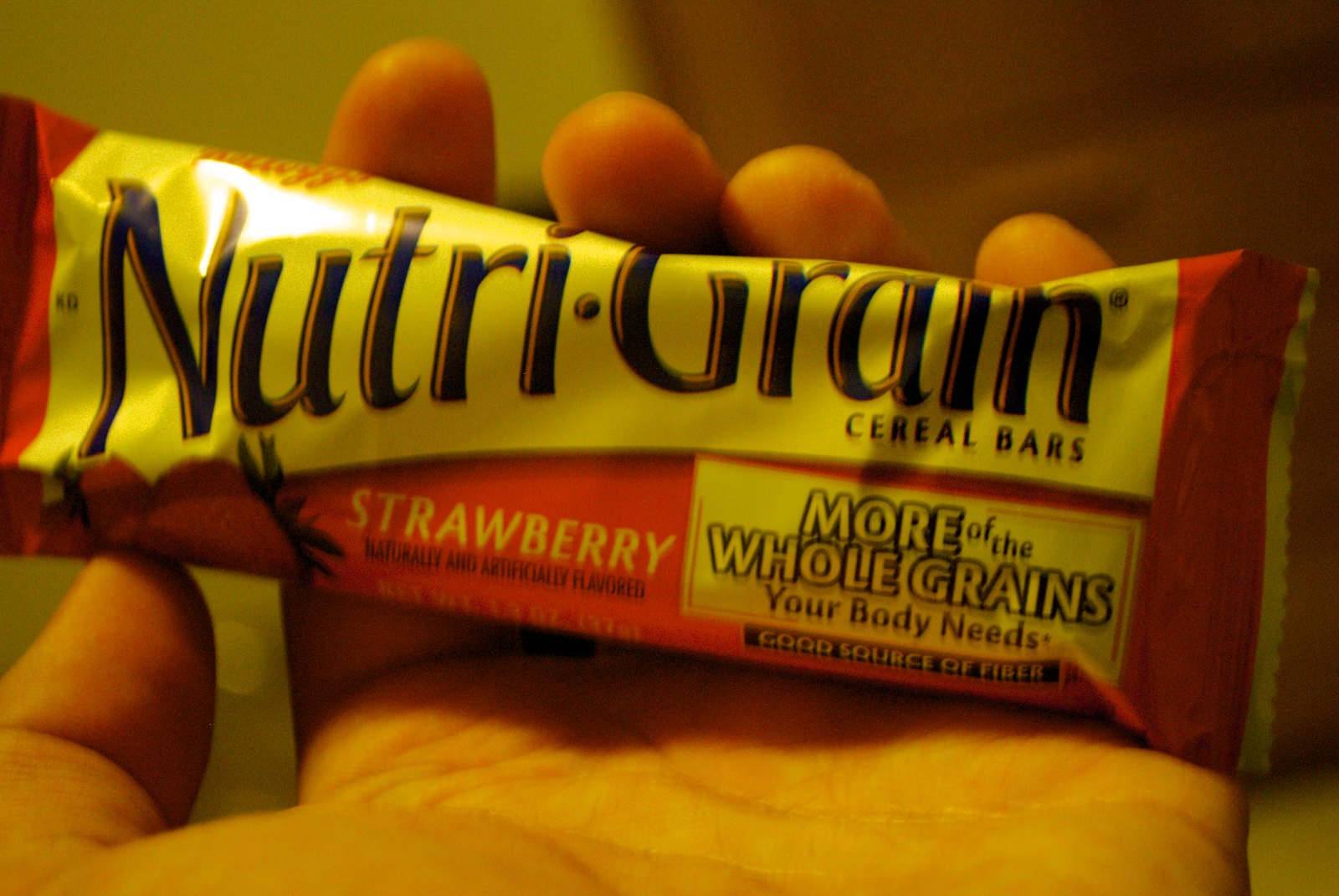The image presents a close-up of a person's left hand holding a Kellogg's Nutri-Grain cereal bar. The packaging primarily exhibits a red and yellow color scheme, indicating it is a strawberry-flavored bar. The main logo, "Nutri-Grain," is prominently displayed in black, fancy font with a gold trim. Above this, the brand name "Kellogg's" is written in red. "Strawberry" is printed in a white or whitish-yellow font underneath the brand name alongside an illustration of red strawberries, and the phrase "naturally and artificially flavored" is noted. A large yellow frame on the packaging advertises "MORE OF THE WHOLE GRAINS YOUR BODY NEEDS" in bold letters, with “GOOD SOURCE OF FIBER” beneath it, both on a black background. The overall image has a yellowish hue, suggesting it was taken under artificial indoor lighting, which casts a yellow tint on not only the packaging but also the person’s hand.